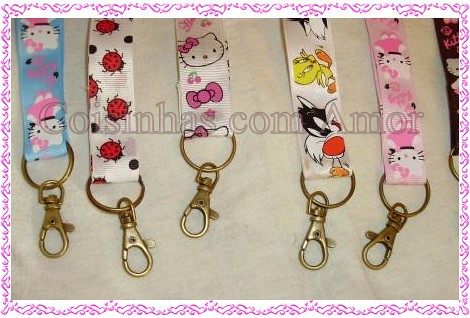The photograph displays six colorful lanyards with brass keyrings and clips, framed by a pink and white border. From left to right, each lanyard has a distinct design: the first is blue with illustrations of white bunnies; the second is white adorned with red ladybugs and black polka dots; the third is white featuring Hello Kitty faces with pink bows and cherries; the fourth is white with images of the Disney characters Sylvester the Cat and Tweety Bird; the fifth is pink with repeating images of Hello Kitty in a pink dress. The final lanyard is light pink and also showcases Hello Kitty in a pink dress. All lanyards share the same style of brass keyrings and clips at their ends.